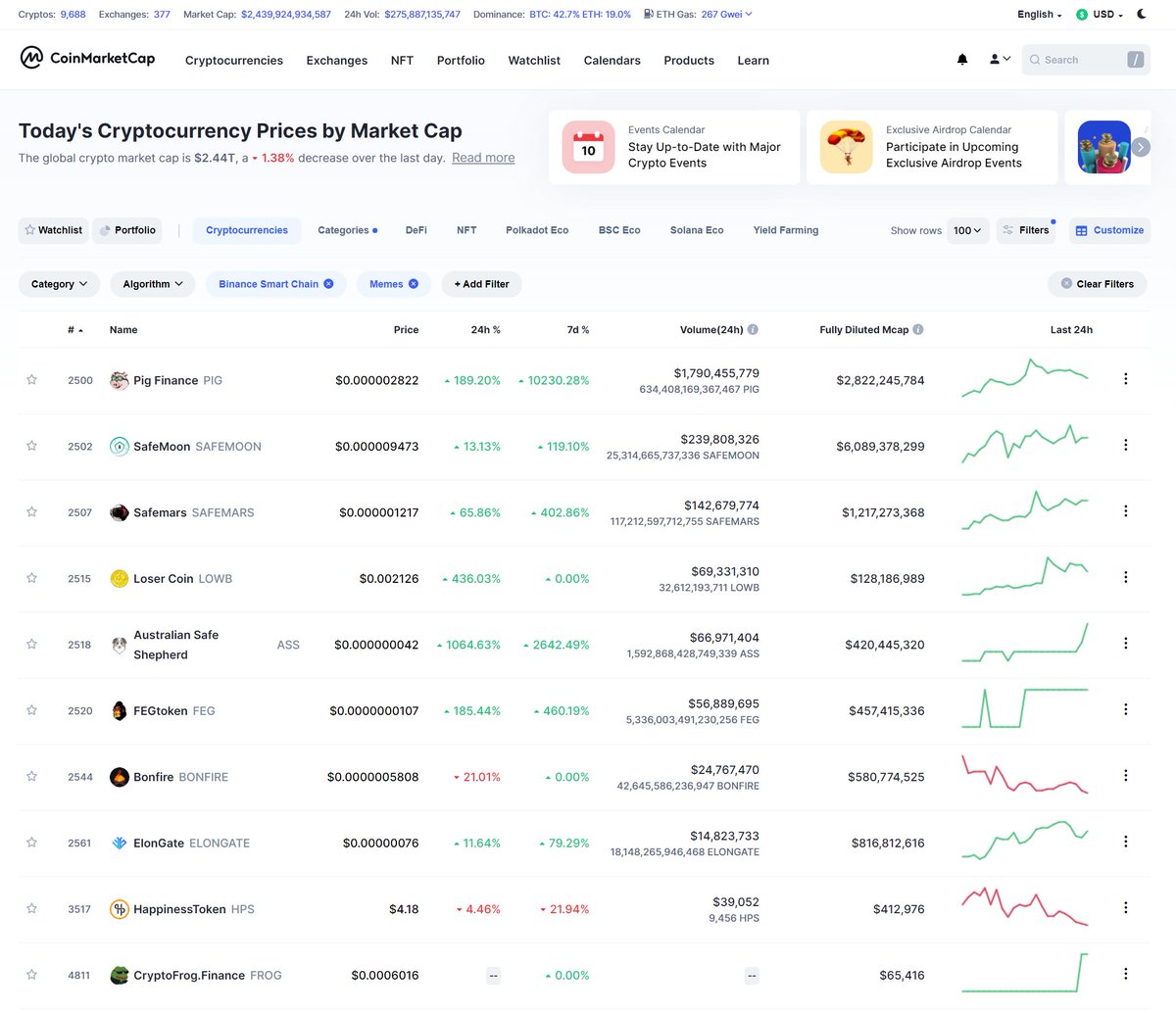The image features a white background with bold text at the top that reads "Cryptocurrency Prices by Market Cap." The content below is an array of cryptocurrency statistics in very small print. Each entry lists the name of a cryptocurrency, its price, the percentage change in the last 24 hours, the percentage change in the last 7 days, the trading volume, the fully diluted market capitalization, and a small line graph illustrating its performance over the past 24 hours.

One detailed example is "Pig Finance," which has a price of $0.000002822. The price has surged by 8,189.20% in the last 24 hours and by 10,233.28% in the last 7 days. The trading volume is $17,179,045,579, and the fully diluted market cap is $2,822,245,784. Similar detailed statistics are listed for multiple other cryptocurrencies.